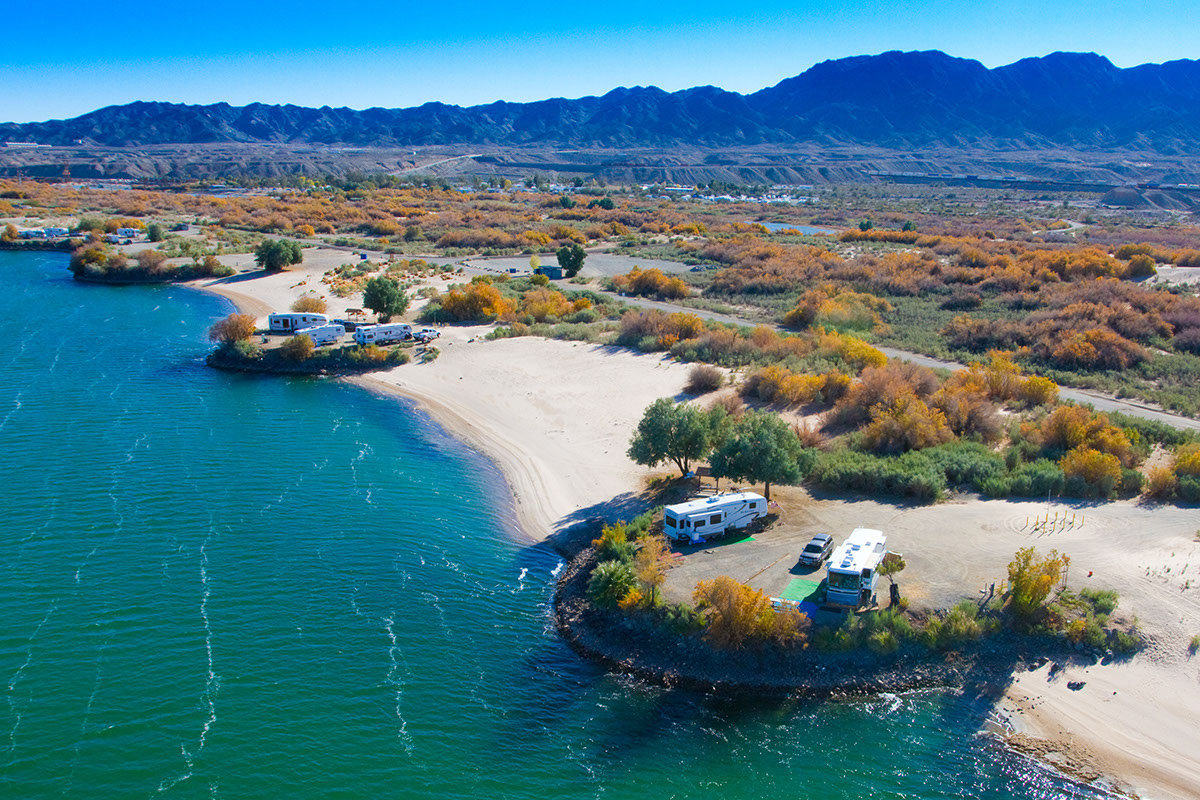This image is a detailed aerial photograph of a picturesque park or camping site set against a backdrop of small mountains. The mountains form a ridge that is taller on the right-hand side and they recede into hills as they approach the foreground, where the terrain becomes flat and covered with a mix of bright orange brush and brownish-green grass. Dominating the foreground is a beautiful blue-green body of water that spans the bottom left diagonal of the image. The water's edge is lined with specially designed camping spots, each marked by semicircular patches of sand or dirt. These spots host several RVs, trucks, and camping equipment, with visible hookups and other amenities for campers. On the left side of the image, the water appears to be part of a lake with a small beach. Trees and bushes of various colors, including yellow, green, and brown, dot the landscape, adding to its vibrant, natural beauty. In the distance, between the elevated viewpoint and the mountains, a small town with various buildings is visible. The sky above is a clear, light blue with no clouds, indicating a sunny day perfect for outdoor activities.